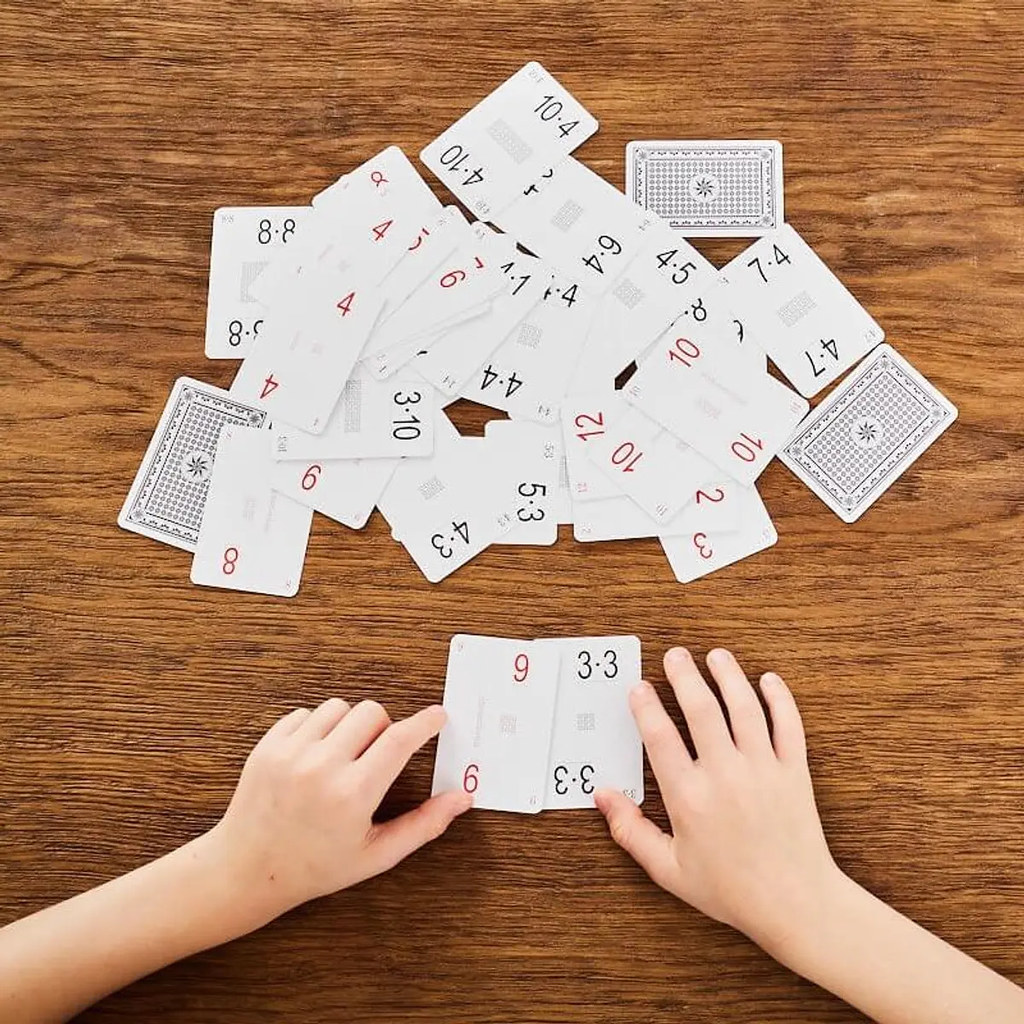In the photograph, we see an indoor setting featuring a child's hands at the bottom of the frame. The child is holding two math cards, one displaying the number '9' and the other showing '3 - 3'. These cards are part of a set used for math practice, where the child matches problems with their corresponding answers. The scattered cards on the wooden table include various numbers and equations such as a red '8', a red '9', '4.3', '5.3', '12', '10', '2', '3', '10', '4.7', '4.5', '6.4', '4.4', '4.1', '9', '5', '4', '4', '8.8', and '4.10'. The reverse side of the cards features a distinctive black and white design. The scene illustrates a young learner engaging in educational activities, likely honing their arithmetic skills through play.